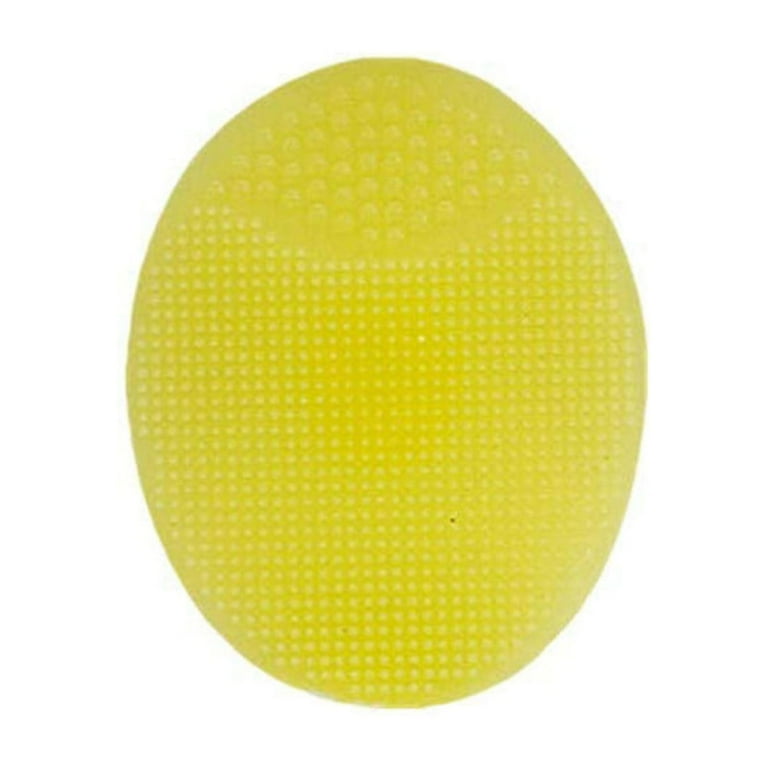This image is a slightly out-of-focus, close-up shot of a yellow silicone face scrubber, egg-shaped with an oval and slightly oblong profile. The background is a uniform white, making the object stand out vividly. The surface of the face scrubber is divided into two distinct textured sections. The lower portion, covering approximately three-fourths of the scrubber, features a consistent pattern of small crosshairs and dots. The top portion transitions into larger, honeycomb-like circles. The scrubber appears slightly greenish-yellow and has a tactile surface ideal for exfoliating. Despite the low resolution and minor blur, the detailed textures are still discernible.